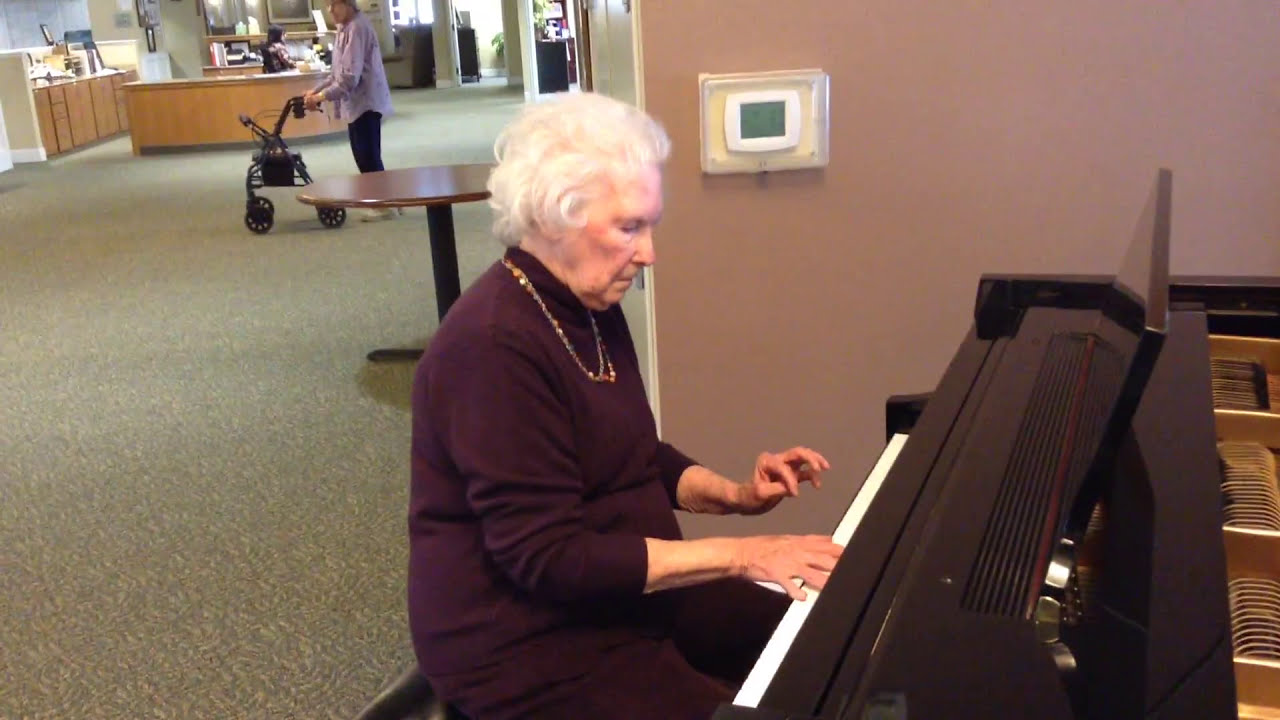An elderly Caucasian woman with short white hair is seated at a brown piano with white keys, playing some notes. She is dressed in a deep purple long-sleeve sweater and matching purplish pants, adorned with a gold beaded necklace around her neck. The setting appears to be an industrial-looking facility, possibly a nursing home, hospital, or clinic, characterized by gray and green carpeting and walls in shades of gray and white. Behind her is a brown half wall with a boxed-in thermostat. The area features several wooden counters, a wood table, and a desk. In the background, another individual, also an elderly woman, is seen using a walker, moving across the room. Further back, there appears to be a reception area with someone seated at a desk and an open door revealing additional light from another room.